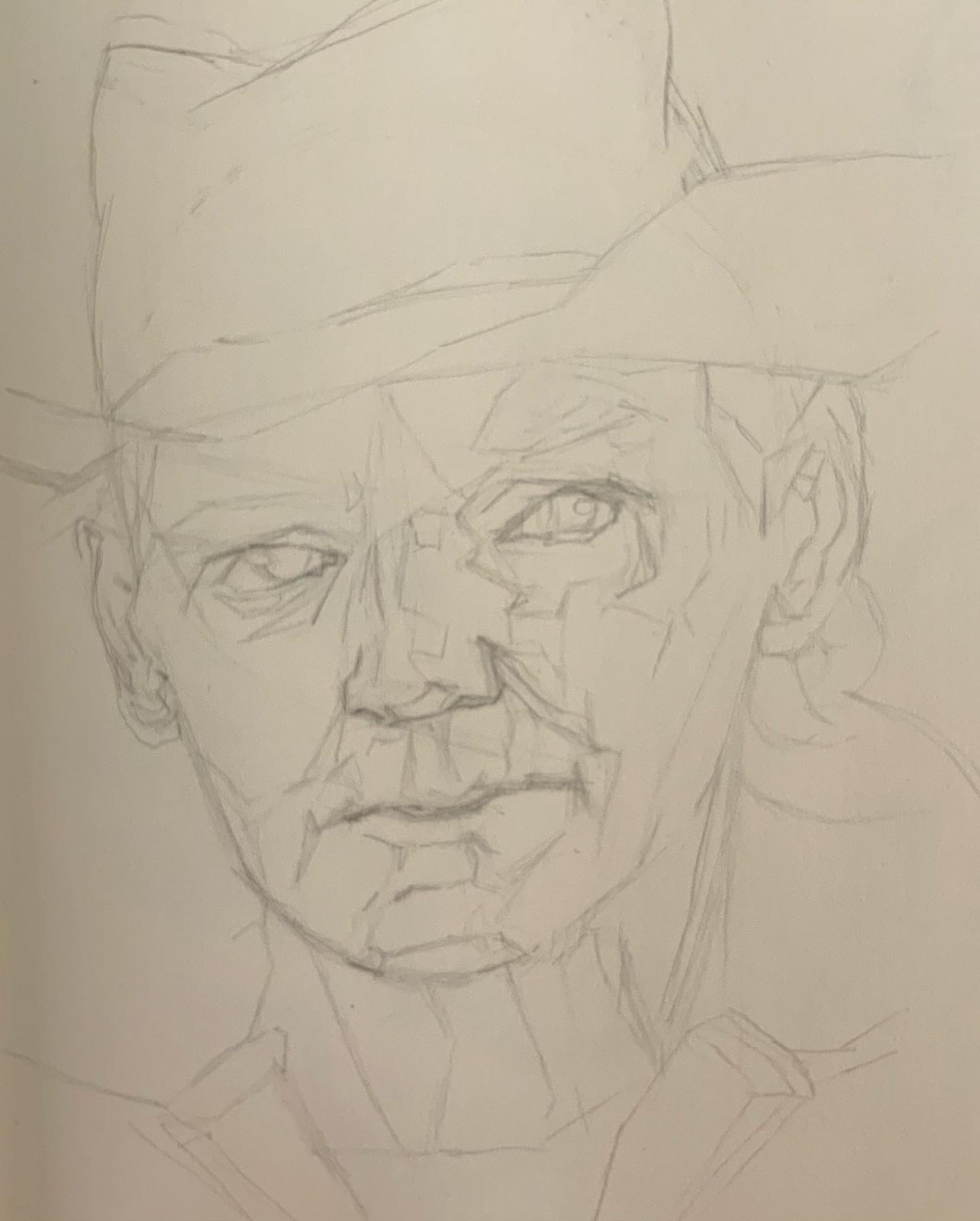This is a pencil sketch on a rectangular piece of light-colored paper that depicts a man wearing a cowboy hat. The drawing is predominantly an outline, with geometric lines evident on the face, likely indicating future shading areas. The man’s face, from the neck up, including part of his shirt collar, is visible. He has a serious expression with a slightly downturned mouth and is looking towards the right of the image with his eyes. His eyes have detailed pupils with a small gleam. The cowboy hat has a distinct, albeit minimally drawn, rim. The image includes detailed features such as the strong jawline, normal nose, and two visible ears. Overall, while intricate in its line work, it is an incomplete sketch, mostly composed of outline lines without shading.